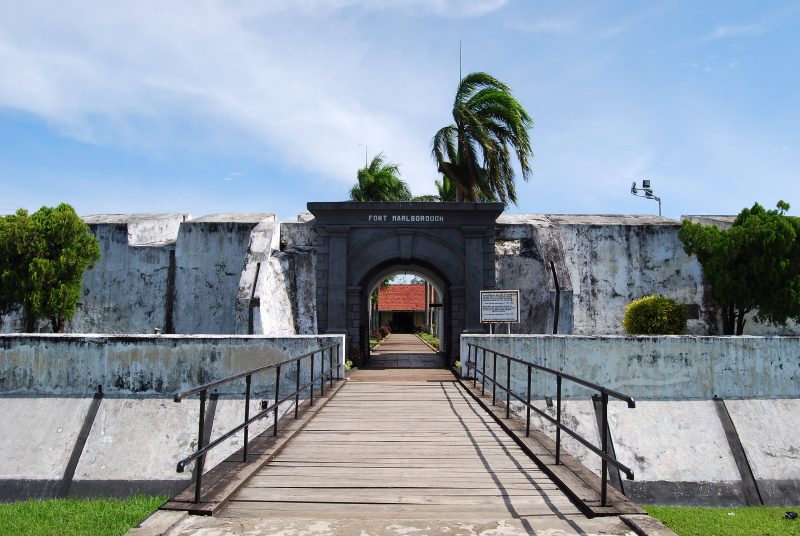The image depicts a weathered, stone structure identified as "Fort Marlboroduch," situated in a southern, tropical region, likely Florida. A wooden walkway spans over a body of water, leading to the arched entrance of the fort, beneath a sign that displays its name. The entrance, shrouded in shadow, invites viewers into the heart of the structure. Encircling the fort are damaged, chipped concrete walls, suggesting neglect and age. In the landscape around the fort, palm trees mingle with evergreen conifers, and grassy lawns stretch on either side of the walkway. Beyond the entrance, a smaller building with a distinct red thatched roof stands out against the blue sky dotted with clouds, hinting at the life within the decaying exterior.